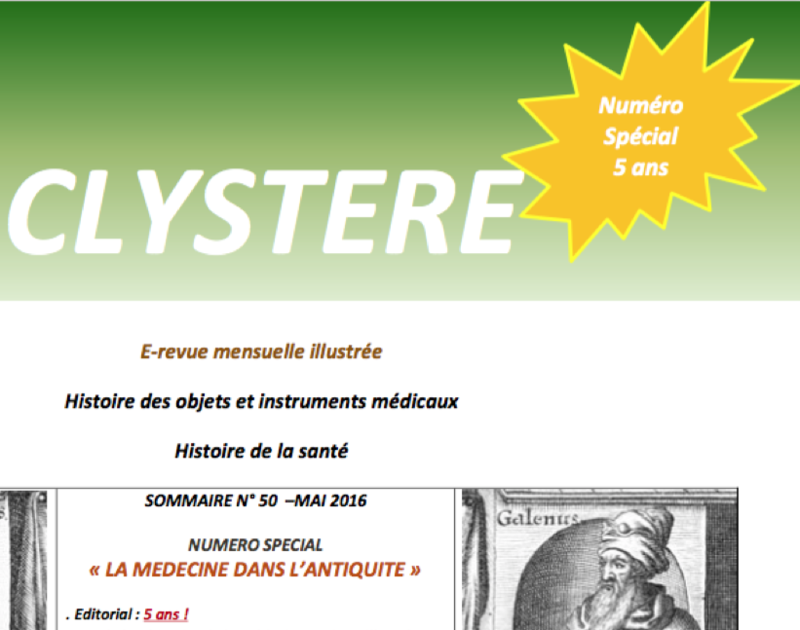The image is an advertisement prominently divided into two main sections. At the top, there is a horizontal rectangular banner featuring a gradient background that transitions from dark green at the top to light green at the bottom. The word "Clystere" is spelled out in large, white text towards the left. To the right of this, within a jagged, starburst-shaped yellow oval, white text reads "Numero Special 5 Ans." Below this banner, against a white background, the text "La Revue Mensuelle Illustrée" is displayed in brown letters. Further below, black text reads "Historia Des Objects Et Instruments Médicaux" followed by "Historia De La Santé." 

At the bottom right of the image is a pencil drawing of an ancient man wearing a turban, sporting a long beard, and dressed in a robe, reminiscent of attire from the 12th to 13th centuries. To the left of this drawing, black text reads "Gal-anis." In the middle section between the drawing and the left side, the text "Sumare Numero 50 Mai 2016 Numero Special: La Médecine Dans L'Antiquité" is displayed. Additionally, there is a mention of "Editorial" followed by "5 Ans!" in red text, highlighting an anniversary. Despite variations in the text across the image, the overall design is rendered in a monochrome palette of black and white, with occasional splashes of red.